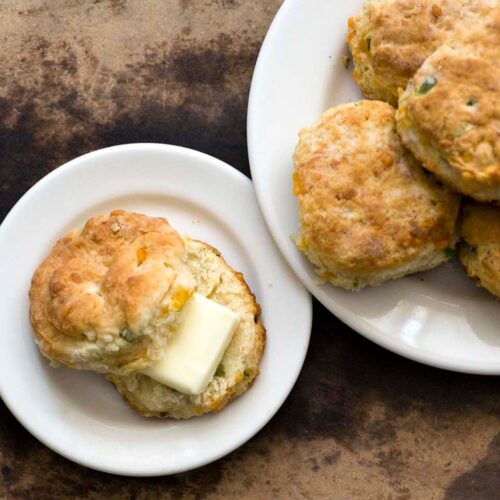The image showcases a marble tabletop with a mix of lighter beige and darker brown areas, conveying an authentic marble appearance. On the bottom left of the photo, a small white plate holds a biscuit that is cut in half. The bottom half of the biscuit features a cube of butter placed on it, square and unspread. The top half of the biscuit is partially covering the buttered bottom half. In the upper right corner, a larger white plate holds a stack of four or five whole, golden-brown homemade biscuits. The biscuits on both plates have a fluffy texture and appear freshly baked, some containing visible green specks and possibly nuts. The tabletop has worn areas, with patches of chipped paint and discoloration, adding texture and character to the background. The scene is detailed with crisp, circular white plates, further emphasizing the rustic and homely atmosphere.